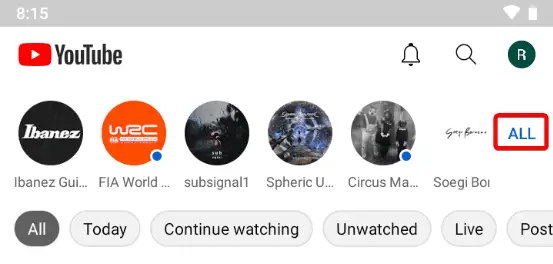This image showcases the YouTube app interface as seen on a mobile device, likely a phone or tablet. At the top, there's a grey status bar displaying the time (8:15) on the left, and the Wi-Fi and battery icons on the right. Below this, on the left-hand side, sits the red YouTube icon with "YouTube" written in black next to it. To the right are icons for notifications, search, and the user profile.

The background of the image is predominantly white. Below the header, several channel icons appear, beginning with "Ibanez" as the first channel, followed by "FIA World," "Sub Signal One," "Spheric You" (with part of the name cut off), "Circus Ma" (with part of the name cut off), and "Soggy Boy." An option to view all subscriptions is available as well.

Further down, there is a row of buttons offering different sorting options: "All," "Today," "Continue Watching," "Unwatched," "Live," and "Posts."